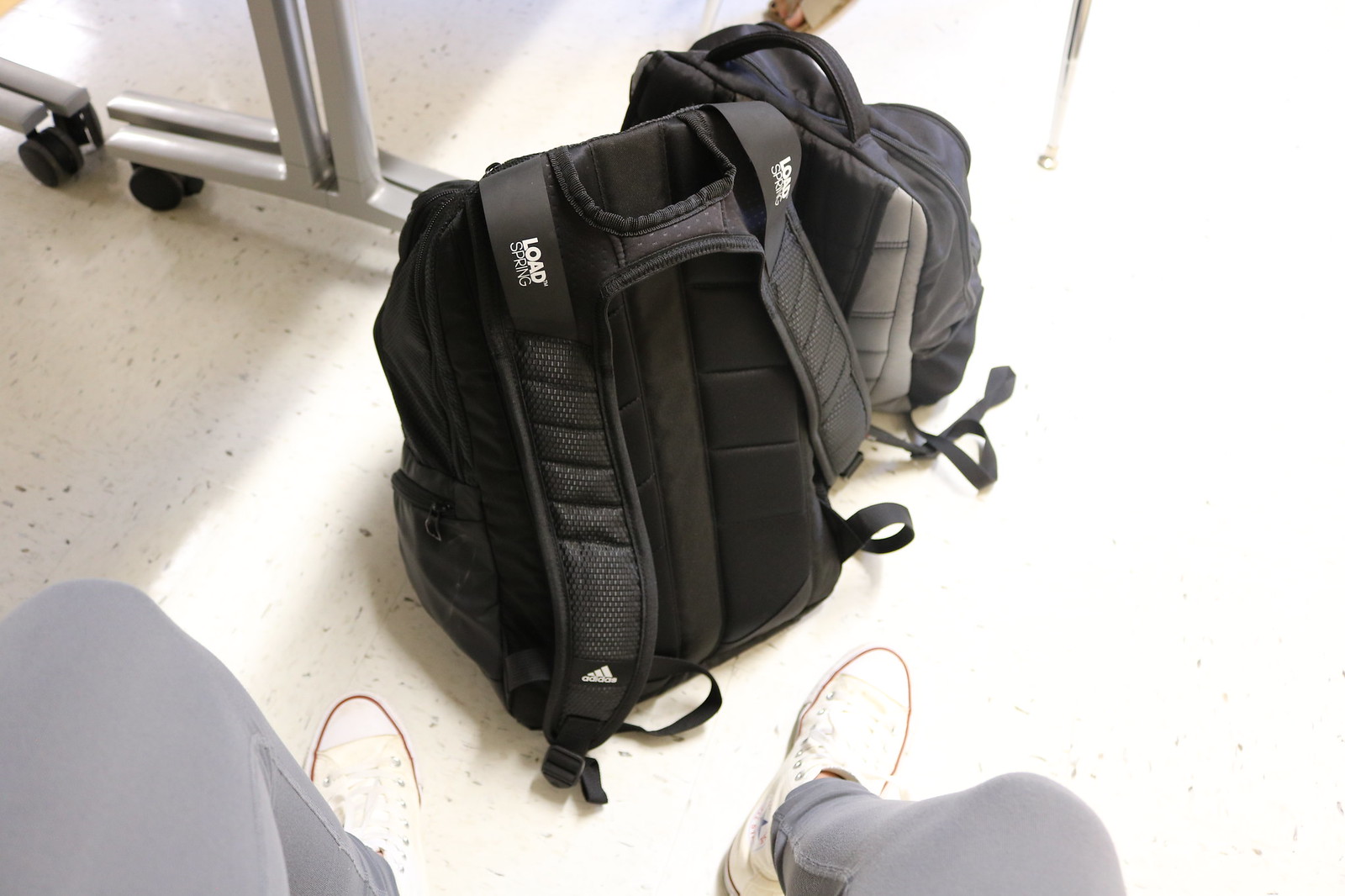A photograph captures the scene from a first-person perspective, likely taken with a cell phone, as evidenced by the visible legs of the person wearing gray sweatpants (or yoga pants) and white tennis shoes (or sneakers) with a red rim. The setting appears to be a well-lit area, possibly an airport or a hotel lounge, indicated by the linoleum floor, which is off-white with dark gray speckles. In front of the person are two sporty black backpacks, each featuring wide soft straps and the Adidas logo prominently visible on the lower left part of one of the straps. The backpacks, which appear to be identical, are situated next to a partially visible metal cart or rolling rack with black wheels.